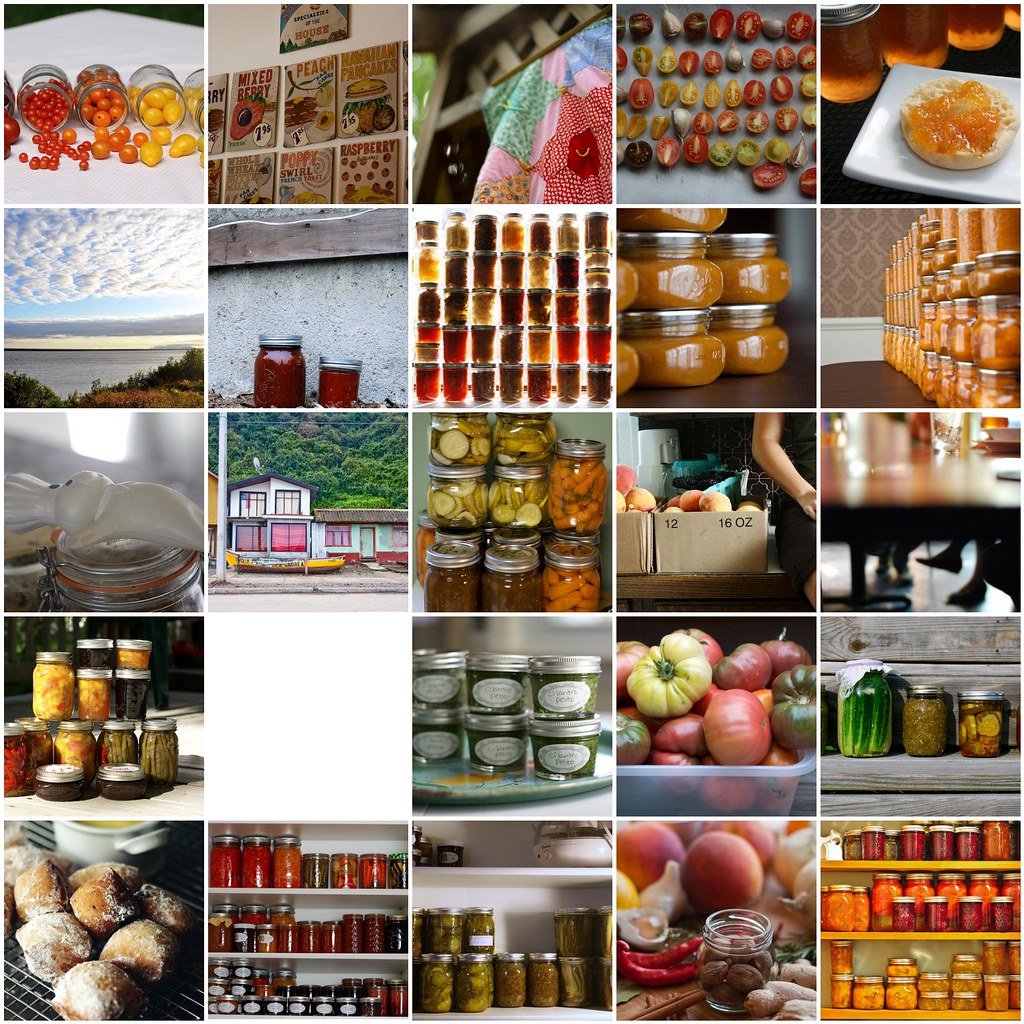The image is composed of 25 equally sized panels arranged in a 5x5 grid, each depicting various food items and a few outdoor scenes. The top-left panel shows jars of colorful cherry tomatoes, and next to it are pictures of fruits and a quilt with vibrant colors. There is a progression of images featuring vegetables, fruits, jams, and jellies, with one panel showing an English muffin. Another row includes a sky scene with clouds, jars filled with a red substance, and a familiar Pillsbury Doughboy figure lying on a jar. Predominantly, the panels showcase an assortment of jarred items, such as pickles and relishes. In the bottom-left panel, powdered scones are visible, while another panel is notably blank and completely white. Interspersed are a few outdoor images, such as a lake with wooden shrubs and a house on a lake shore with a small boat. The scenes, rich in colors ranging from tan and orange to deep maroon red, form a vivid collage mostly of food items, with 22 panels focusing on various jarred fruits, preserves, and baked goods, and two panels displaying serene outdoor visuals.